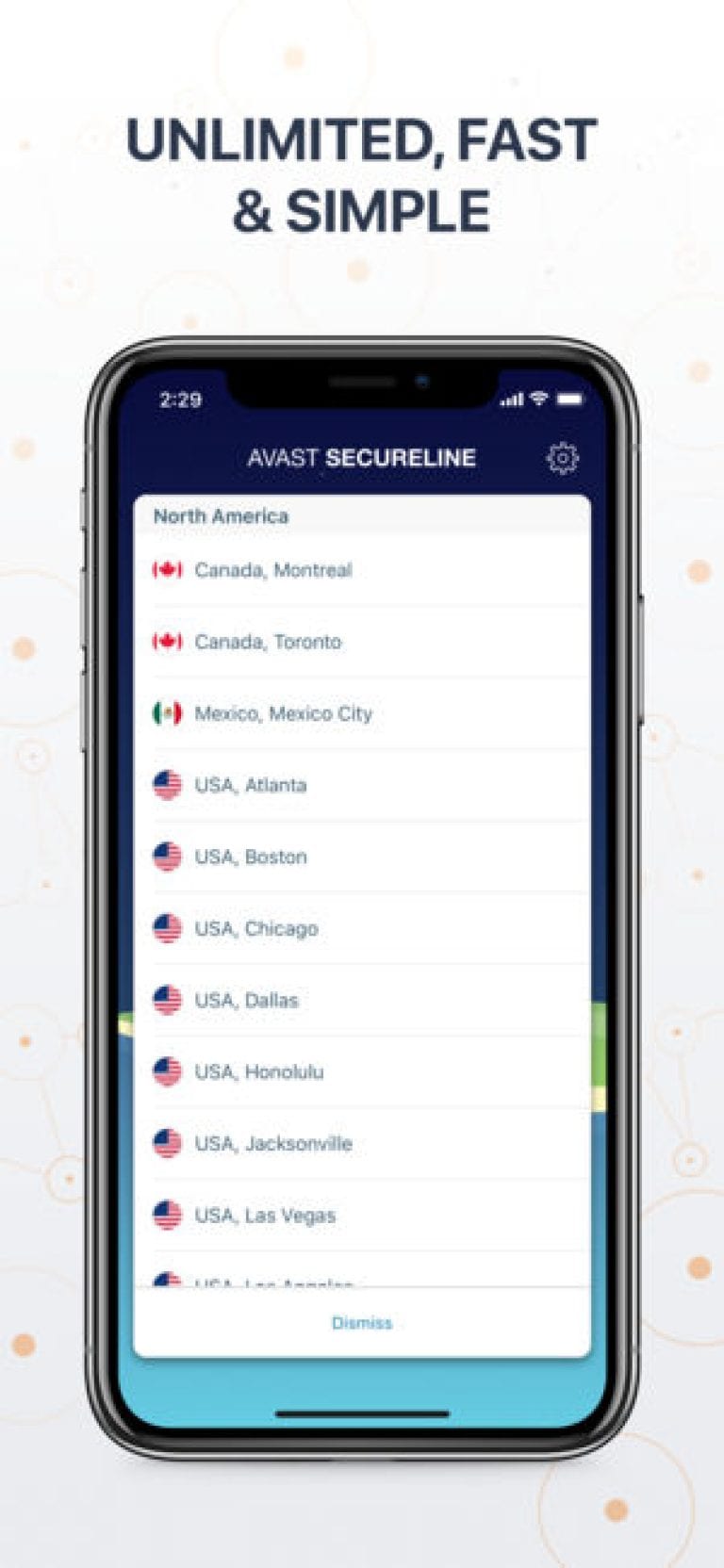The image features a cell phone screen prominently displaying a list of cities and corresponding country flags. At the top of the screen, in bold blue letters, are the words "Unlimited, Fast, and Simple." The time shown in the upper left corner of the screen is 2:29, and next to it, various icons indicate battery life and signal strength. 

Below these icons, the screen displays the header, "A Vast Secure Line," with an option symbol to its right. Under the header, the list is organized by region, beginning with "North America" in black letters. The cities and countries listed beneath include:

- **Canada, Montreal** with a Canadian flag
- **Canada, Toronto** with a Canadian flag
- **Mexico, Mexico City** with a Mexican flag
- **USA, Atlanta** with an American flag
- **USA, Boston** with an American flag
- **USA, Chicago** with an American flag
- **USA, Dallas** with an American flag
- **USA, Honolulu** with an American flag
- **USA, Jacksonville** with an American flag
- **USA, Las Vegas** with an American flag

At the bottom of the screen, in blue letters, is the option to "Dismiss."